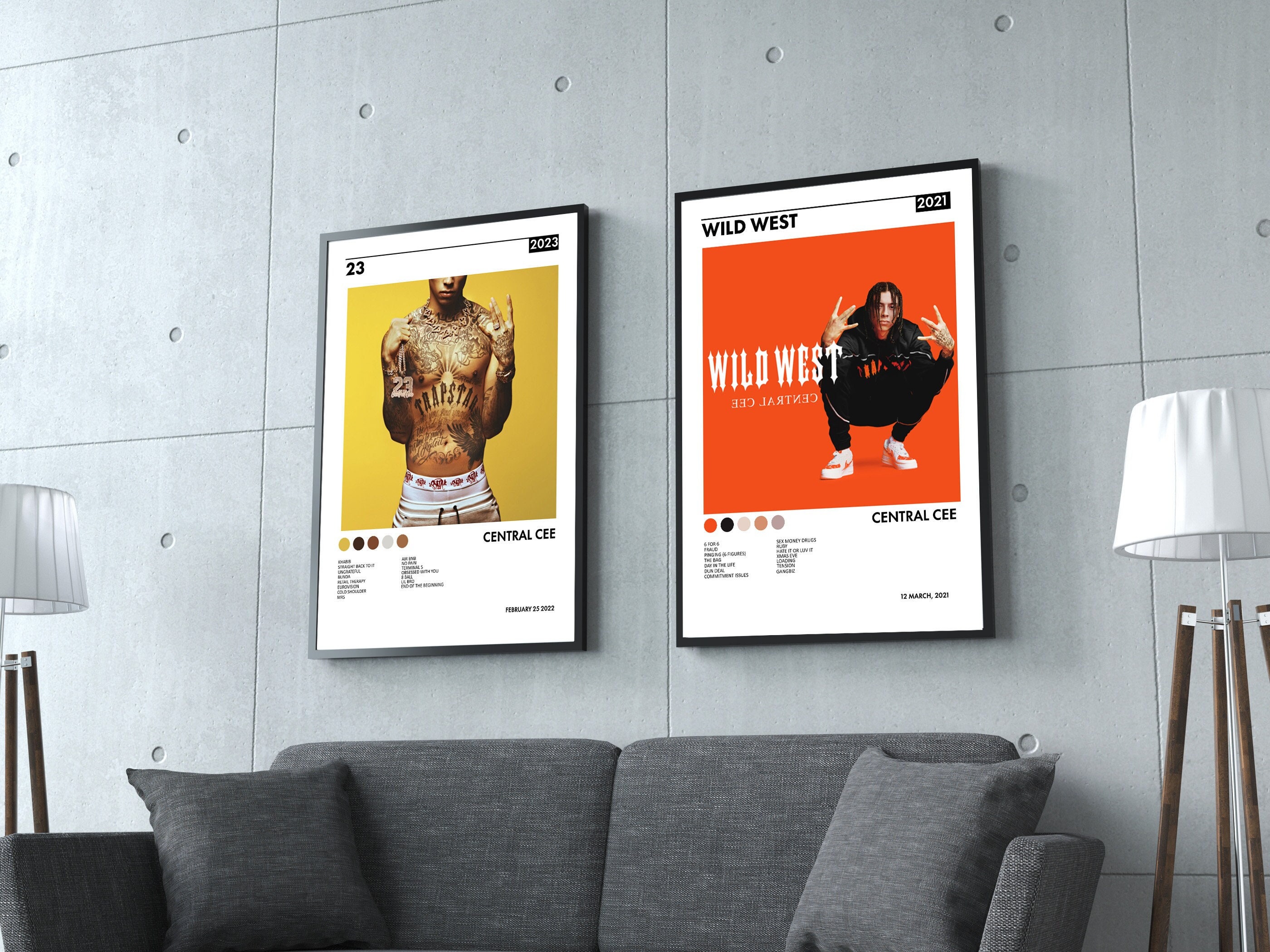This photograph captures a modern apartment interior centered on a cozy, gray sofa with two plush back pillows and two accent pillows at each corner. Above the sofa, two stylish posters on a gray-tiled wall command attention. The left poster features a heavily tattooed man with the text "23," "2023," and "Central C" along with a February 25th, 2022 date, suggesting it might be an album cover. The right poster, with an orange background, depicts a lighter-skinned man with dreads in a Siberian squat position, titled "Wild West" and "Central C," dating to 2021, indicating it is likely from the same artist. Flanking these posters are two tall lamps with slender wooden legs and white circular shades, adding a touch of elegance to the modern décor. The overall color scheme is sophisticatedly monochrome with the striking yellow and orange hues of the posters providing vibrant contrast, making the entire setting both clean and visually appealing.